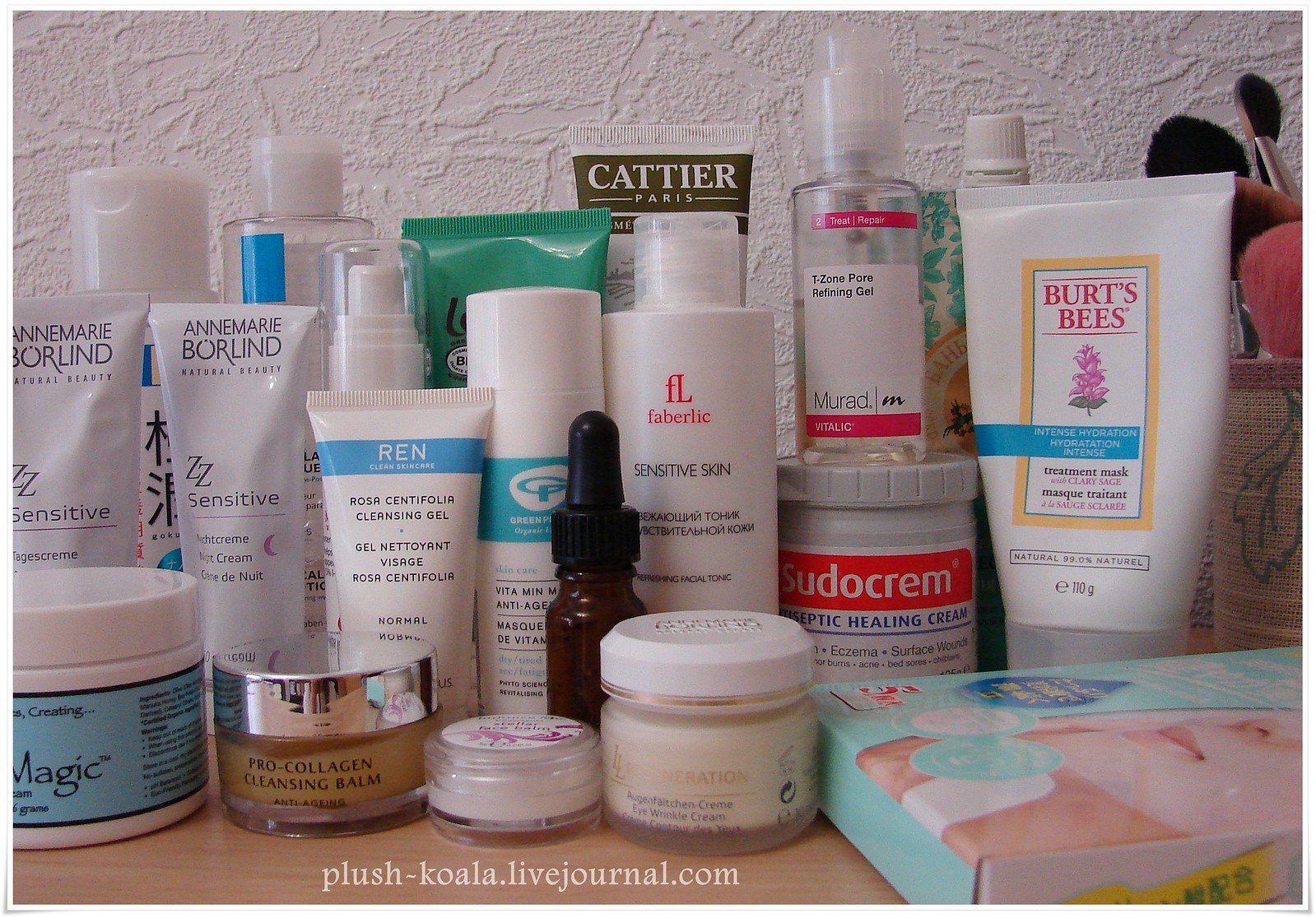A detailed photograph showcases an array of facial products and skin creams, neatly arranged on a light wooden, Formica-style surface. In the bottom corner of the image, white text reads "plush-koala.livejournal.com." The assortment includes numerous tubes displayed upside down, several small spray bottles, and jars, each adorned with various labels.

Prominently featured is a white tube with a blue stripe, labeled "REN Clean Skincare" with accompanying black text that reads "Rosa Centifolia Cleansing Gel" along with additional French writing. Below this, a small glass bottle with a shiny chrome top is identified as "Pro-Collagen Cleansing Balm." To the right, a squeeze bottle is labeled "Burt's Bees Treatment Mask" with details including "Clark Sage," "110 grams," and "natural 99.0% Naturel." The surface teems with a diverse collection of skincare items, highlighting an extensive range of treatments and cleansers in various forms and packaging.